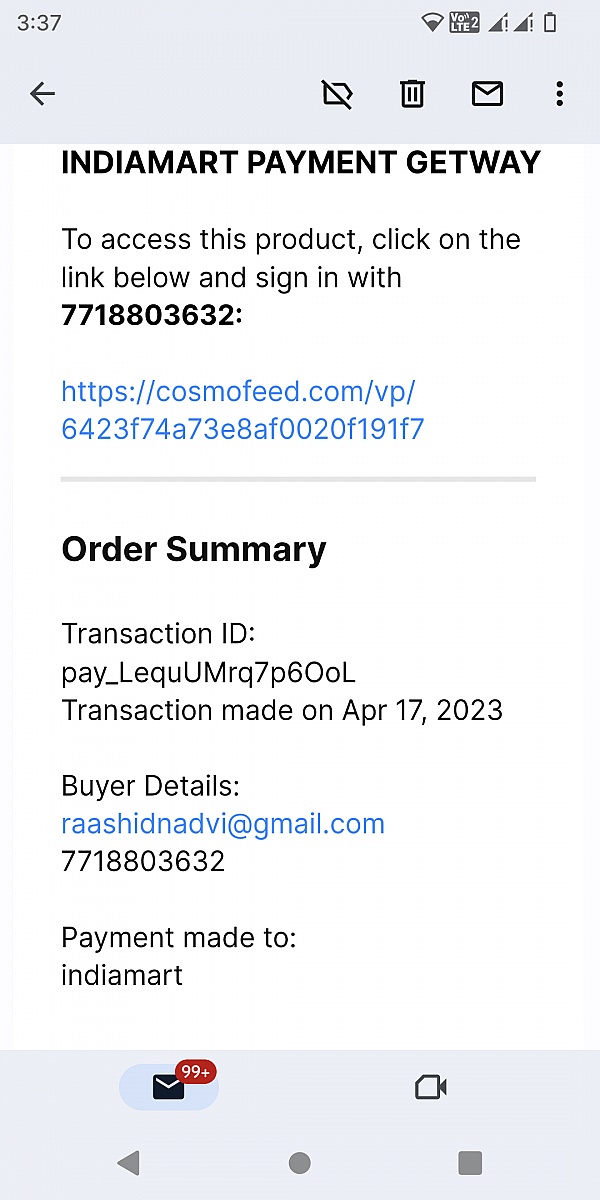This image depicts a smartphone screen displaying an email. At the top of the screen, the time is shown as 3:37, accompanied by various status icons in the top right corner, including Wi-Fi strength, an LTE indicator, and an empty battery symbol. The top section of the screen has a gray background.

Directly beneath the time display, there are several icons: a left-pointing arrow for navigation, an icon resembling a tag with a line through it, a trash can icon for deletion, an envelope symbol, and a menu represented by three dots.

The email content itself is displayed on a white background. The subject line reads "India Mark Payment Gateway" in bold letters. The email instructs the recipient to access a product by clicking on the provided link and signing in with the number 771-880-3632. The link given is "https://cosmofee.com/vp/6423F74873E8AF0020F191F7".

Below the link, there is a header labeled "Order Summary" in bold letters, followed by the transaction details:

- **Transaction ID:** K_LEQUMRQ7P6O60ROOL
- **Transaction Date:** April 17, 2023
- **Buyer Details:**
  - Name: Rashid Nadvi
  - Email: RashidNadvi@gmail.com
  - Phone: 771-880-3632
- **Payment made to:** India Mark

At the bottom of the phone screen, there is another gray section containing an email button with an envelope icon and a notification badge showing "99+" in red. Standard navigation buttons are also visible: a triangle pointing left, a circle, and a square.